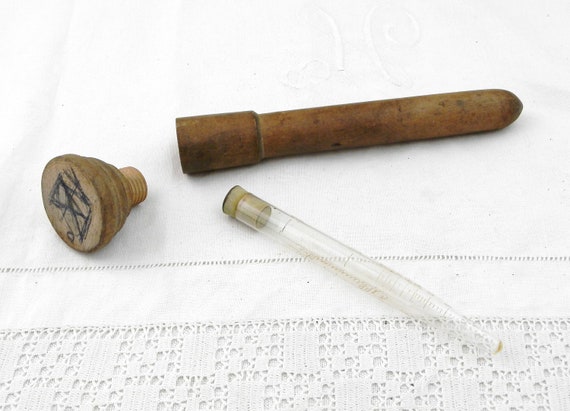In the photograph, a cork stopper with scratched or etched ink and another elongated rectangular cork stopper are positioned side-by-side. Below them is a long, thin glass tube resembling a test tube, indicative of older chemistry instruments. These items rest on a white tablecloth featuring a unique, quilted stitched pattern. The first cork has some markings that look like initials, possibly "DP". The wooden components include a cigar-shaped tube with a hemispherical cap that screws on, perhaps serving as a protective case for the glass tube. The realistic, horizontally oriented image, devoid of text, captures these eclectic objects against the intricately patterned white cloth, evoking a sense of antique laboratory equipment.